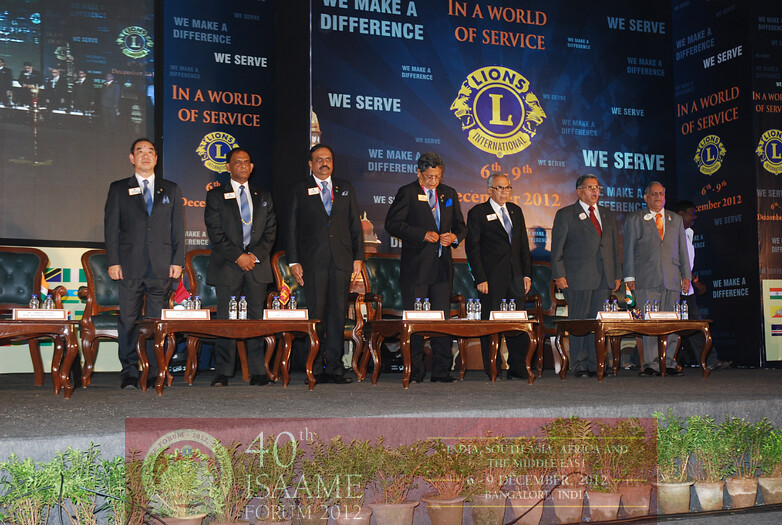In the image, seven men dressed in suits, ties, and white shirts stand formally on a stage, suggesting a sense of occasion. Each man wears a name badge, indicating their official capacity. The stage is set with green cushioned wooden chairs and wooden tables, each table adorned with bottles of water. Behind the men, a prominent LED screen displays the logo and messages of Lions International, including phrases like "We serve. We make a difference." The scene is part of the 40th ISAAME Forum 2012, as indicated by a banner at the base of the stage. The setting is further decorated with multiple potted plants arranged along the stage, adding a touch of greenery to the formal atmosphere. Off to the side, additional chairs suggest other participants might be present but out of view. The men appear to be either being introduced or reciting a pledge, contributing to the formal and ceremonial nature of the event.